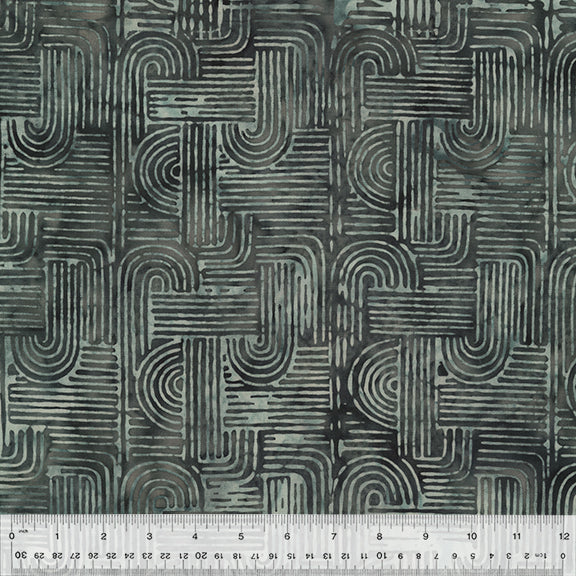This photograph depicts a detailed repeating pattern reminiscent of vintage 1970s graphic design, possibly seen on wallpaper or fabric. The intricate design features a series of geometric shapes—square shapes with rounded corners, upside-down L shapes, J shapes, and rectangles—formed by alternating white and thicker black lines. The shapes are interconnected with semi-circled curves creating a woven appearance, further enhanced by a marbled texture in dark forest green, lighter greenish-teal, and blue hues. These patterns occupy three complete rows before being partially overlaid by a semi-transparent, standard 12-inch white ruler at the bottom of the image. The ruler showcases measurements up to 12 inches alongside an upside-down scale from 0 to 30 centimeters, offering a glimpse of the patterned design beneath it. The detailed depiction and slight imperfections suggest the pattern might have been created using techniques like batik, adding to its artisanal and tactile quality.